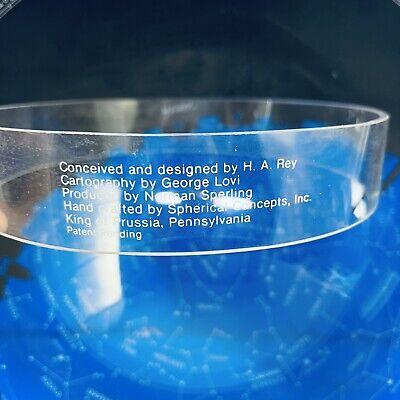The image depicts a highly zoomed-in, clear circular object, likely made of glass or plastic, approximately an inch and a half thick. This transparent object features detailed etching and engraved text that reads: "conceived and designed by H. A. Ray, cartography by George Lovey, produced by Norman Sperling, handcrafted by Spherical Concepts Inc., King of Prussia, Pennsylvania, patent pending." The object hovers over a bright blue surface, possibly a table or paper with white lines drawn on it. The background displays a gradient of bluish, blackish, and gray hues, appearing out of focus and adding an enigmatic ambiance to the image. The object is illuminated, capturing reflections and highlights which suggest careful lighting. Despite the clear view of the text and object, its exact purpose remains unclear, potentially hinting at a scientific or specialized tool.